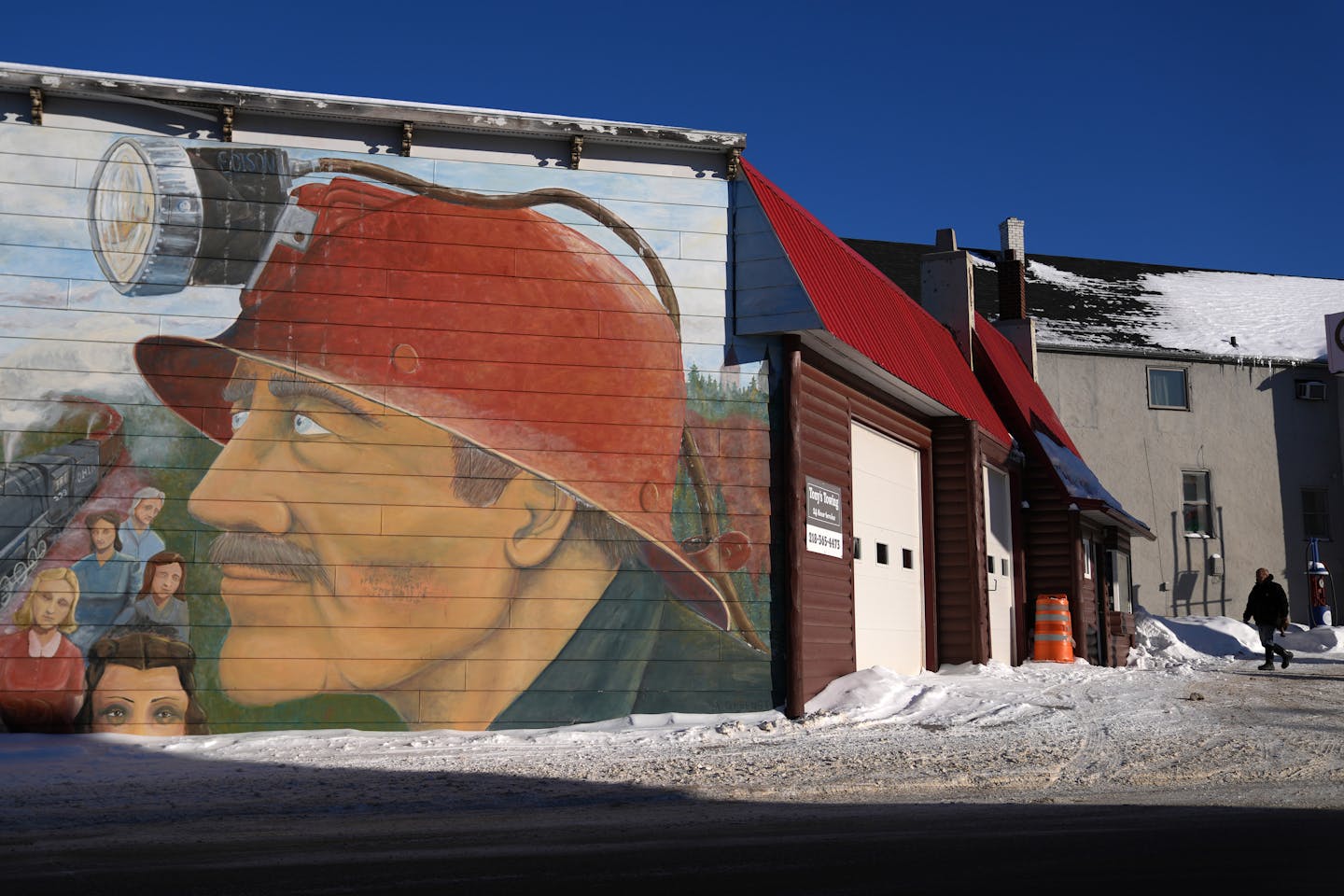The image depicts a snow-covered urban scene featuring a building with two garage doors on its front right section, suggesting it might be a garage or shop. On the left side of the building, a detailed mural is painted on brick, prominently displaying an older man with a mustache wearing a red hard hat with a headlamp, suggestive of a firefighter or railroad worker. Surrounding the man's larger-than-life face are five smaller figures, seemingly all women, positioned to his left, accompanied by the image of a train on tracks. The scene is set in a slushy, snow-laden environment with plowed snow accumulated nearby. An orange construction cone sits in front of the garage, and another building, gray with snow on its roof, stands to the right. In the background, a bundled-up man walks between the buildings, adding to the impression of a cold, wintry day.